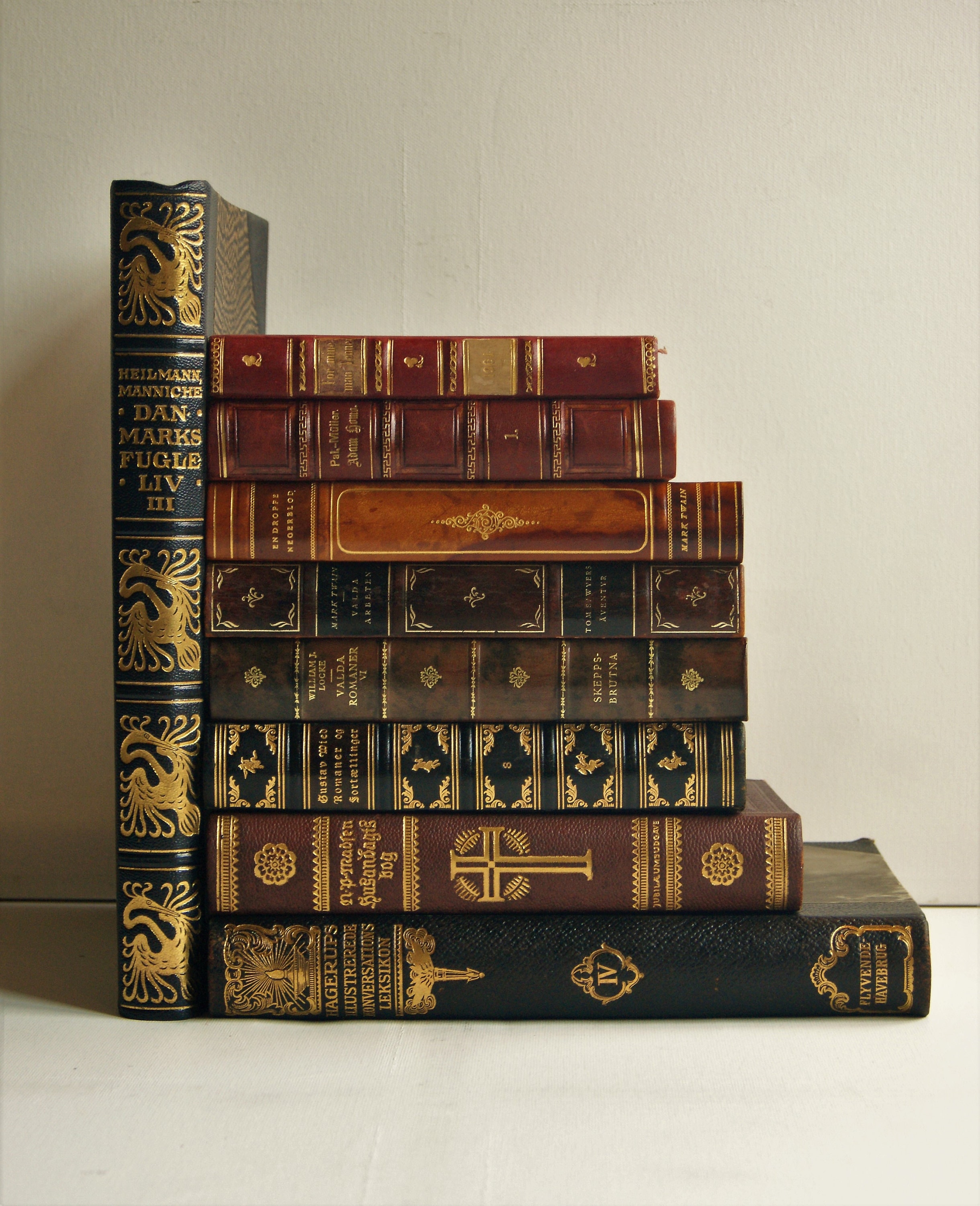This photograph captures an array of aged, leather-bound books arranged on a pristine white shelf against a white background. Dominating the left side, a tall, upright book features a blue cover with golden embossing, displaying names such as Heilman, Maniche, Dan, Marks, and Fugel. Next to it, a stack of eight books lies horizontally, creating a visually appealing gradient from the largest book at the bottom to the smallest on top. These books, characterized by their old-fashioned appearance, vary in color from dark blue, brown, and reddish-brown, to maroon, with intricate gold embellishments adorning their spines and covers. The bindings evoke a sense of historical significance, akin to ancient tomes or classic literature, with the text in gold being largely illegible. This meticulous arrangement of books forms an L-shape, with the volumes in varying sizes and shades, collectively illustrating a rich tapestry of literary antiquity.